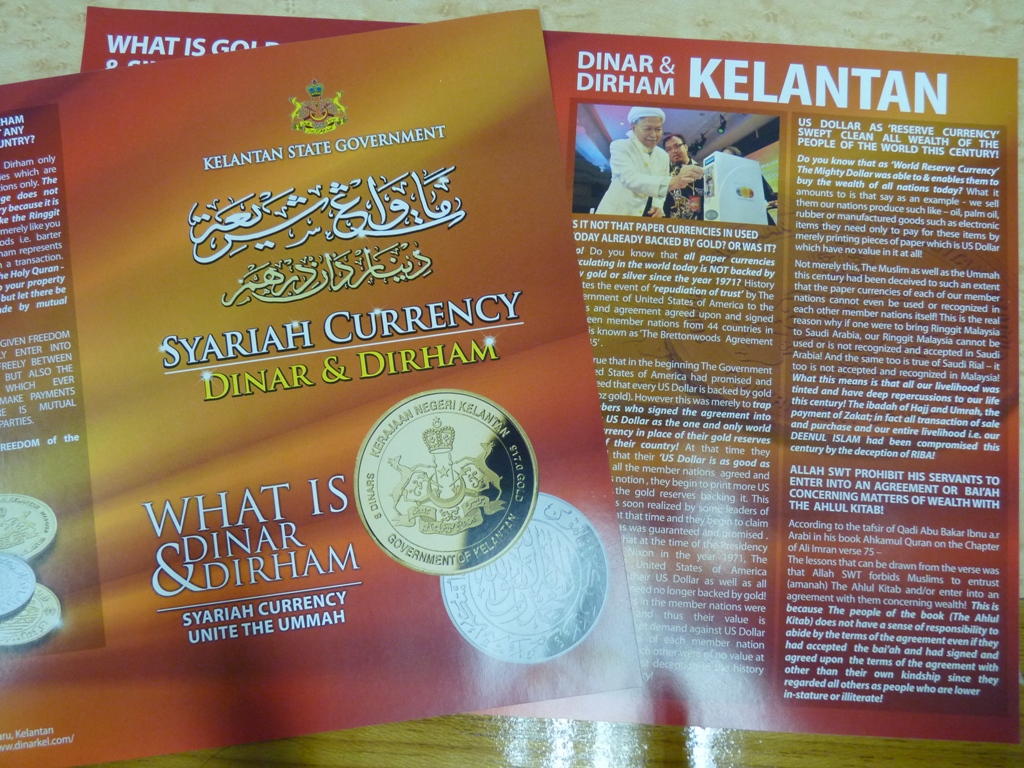The image showcases a glossy brochure laid out on a wooden table, prominently displaying information about the Kalinten State Government's Syrian currency, specifically the dinar and the dirham. The dominant colors of the pamphlet are reds, yellows, and oranges, adding vibrancy to the presentation. The front cover of the brochure features the text "Kalinten State Government" and "Syrian Currency: Dinah and Dirham," along with the slogans "What is Dinah and Dirham?" and "Unite the Ummah." A set of pictures of one gold and one silver coin accompanies the text. The back or inside of the brochure provides detailed paragraphs about the significance of the dinar and dirham, emphasizing how the U.S. dollar as a reserve currency has swept the wealth of people globally. Also depicted is an image of a person in a white jacket with a furry collar, appearing to place the currency into a slot. Arabic writing is seen on the front, enhancing the cultural context of the content.